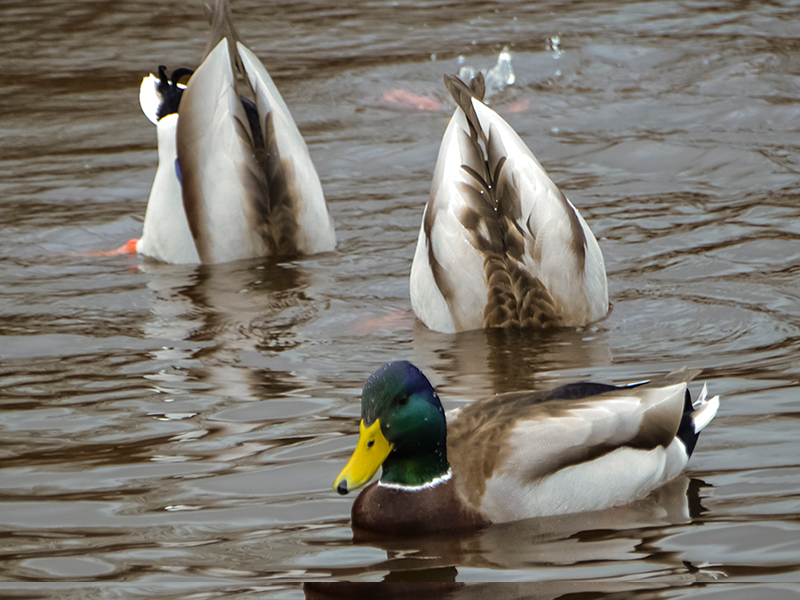In an outdoor setting during daylight, the image features three ducks floating in water that appears brownish-gray. The duck at the bottom center of the image faces the camera directly, displaying a head that is bright green or dark blue with a yellow beak and a distinctive white ring around its neck. This duck's body feathers are a mix of white, brown, and black. In the background towards the center, two additional ducks are visible, showing only their backs as they face away from the camera. Their bodies are similarly colored in white and brown. Additionally, towards the far end of the image at the top, another duck is partially submerged, creating splashing bubbles as it dives deeper into the water. Ripples and waves are visible on the water's surface, adding dynamic texture to the scene.